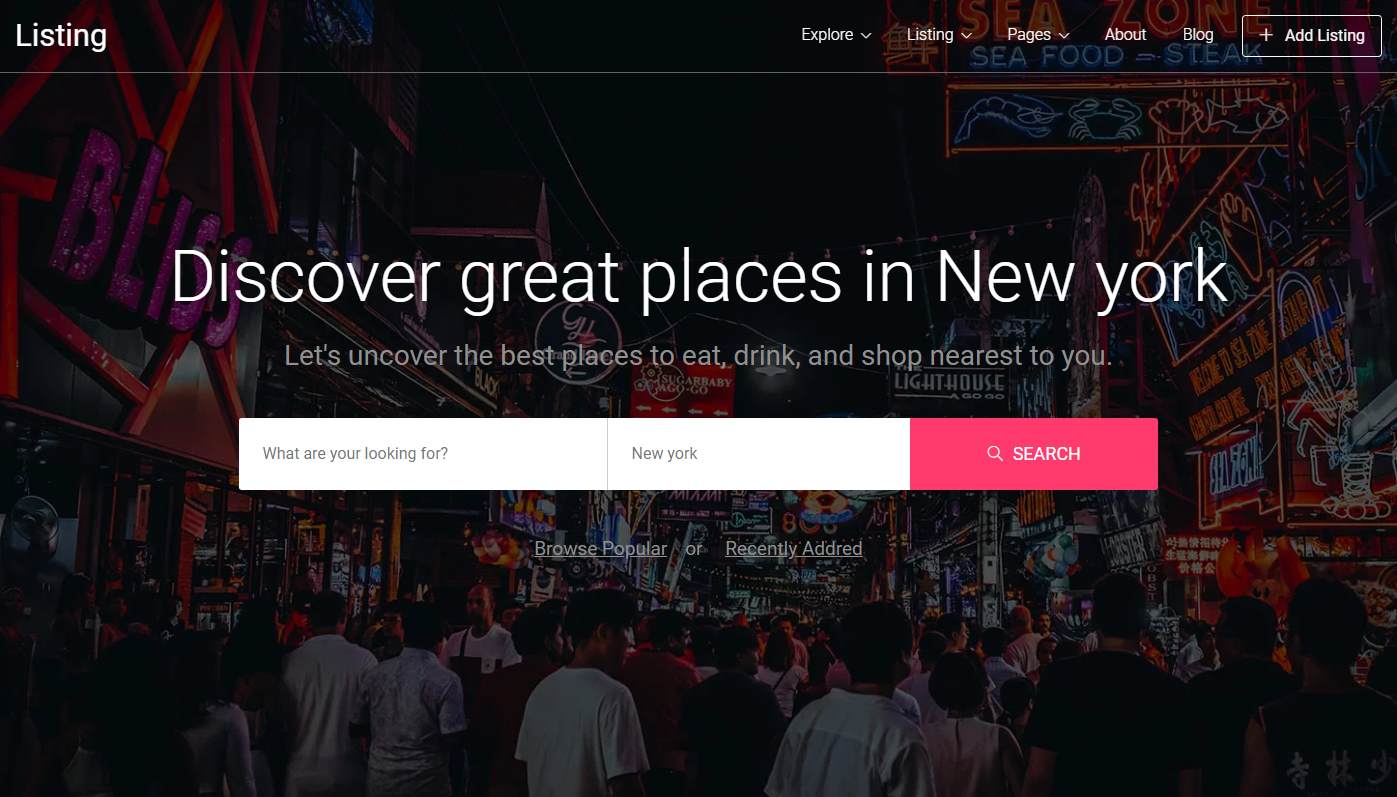The image resembles an advertisement for a website dedicated to discovering various locations in New York City, including shops, restaurants, and bars. The horizontally-oriented rectangular image features a nighttime street scene in New York, bustling with illuminated signs and vibrant lights from numerous establishments. Pedestrians are seen walking down the street or sidewalk toward the bottom center of the image, adding a lively urban feel.

In the top left corner, the word "Listing" is prominently displayed. Centrally, bold text reads, "Discover great places in New York. Let's uncover the best places to eat, drink, and shop nearest to you." A large search bar dominates the middle of the image. The left side of the search bar is white with text prompting, "What are you looking for?" beside a box indicating the location, New York. The right side is highlighted in red, featuring a magnifying glass icon, inviting users to start their search.